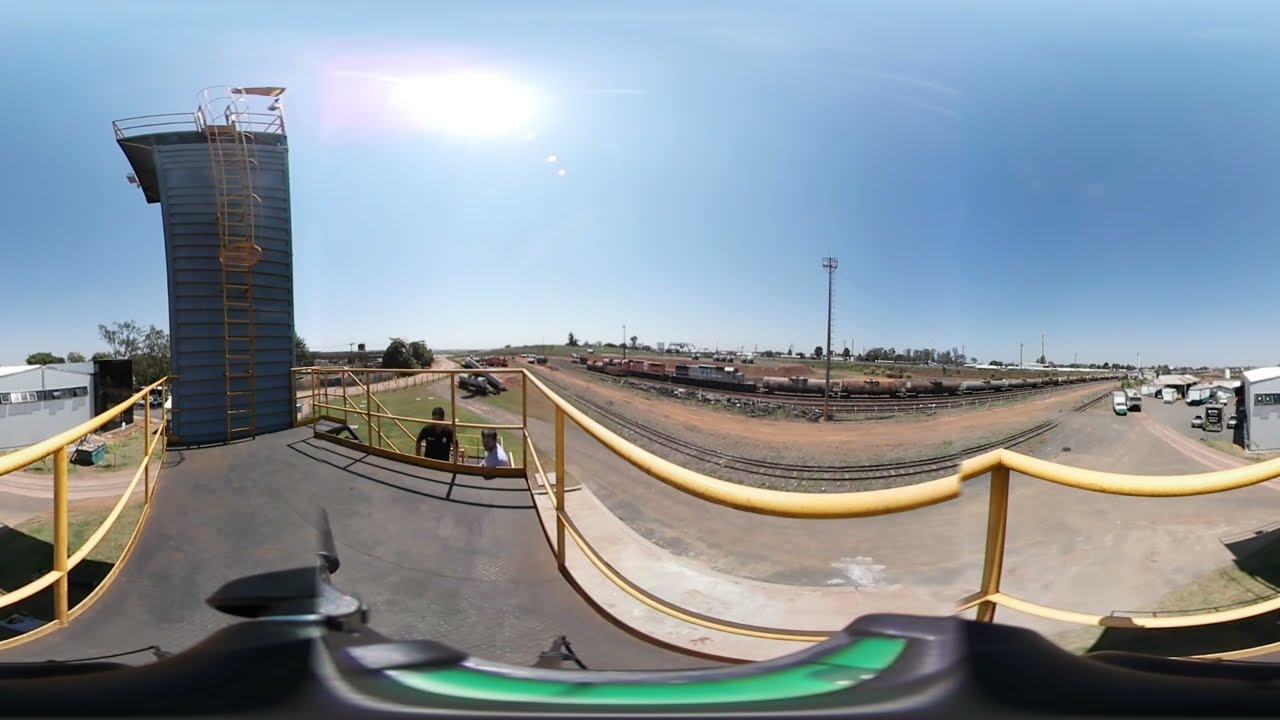This horizontally aligned rectangular image, bordered by thick black lines at the top and bottom, captures an outdoor scene under a clear blue sky with a few wispy white clouds. The sun, appearing as a bright white blob, is positioned in the upper central part of the picture. Dominating the left side of the image is a tall, gray metal structure with a yellow ladder affixed to its side, likely serving as a lookout tower. This tower is surrounded by a yellow metal railing that encloses a concrete walkway.

Below the walkway, near the centered yellow railing, are two individuals: one dressed in black and the other in white, seemingly engaged in conversation. To the right of the image, a train navigates a curve on a paved track, accompanied by a series of trucks and a smaller gray building with a white roof in the distance. Below the people, at the very bottom of the image, part of a black plastic object with a green center is visible, possibly the top of a motorcycle. The entire scene suggests an industrial area, perhaps a racetrack or train lot, providing a vivid snapshot of both human activity and infrastructure.